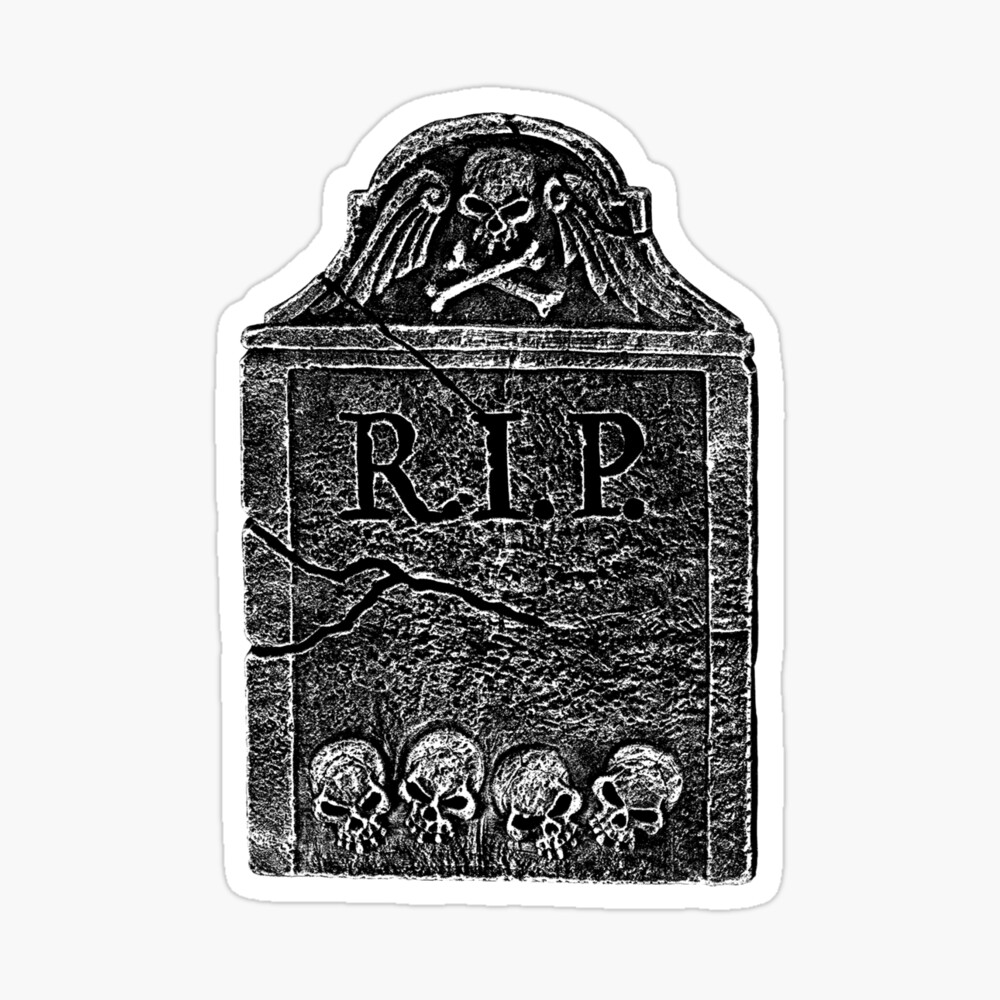The image depicts a detailed black-and-white sticker or decal of an old, cracked headstone. The headstone, outlined in white with a subtle gray drop shadow, stands against a nearly white background. Its top part is arched with a bell shape, featuring a central skull and crossbones flanked by angel wings on both sides. The engraving "R.I.P." is prominently displayed at the top of the headstone. The base of the headstone bears carvings of four skulls aligned side-by-side, adding to the eerie and intricate design. The weathered look and cracks running through the tombstone enhance its aged appearance.